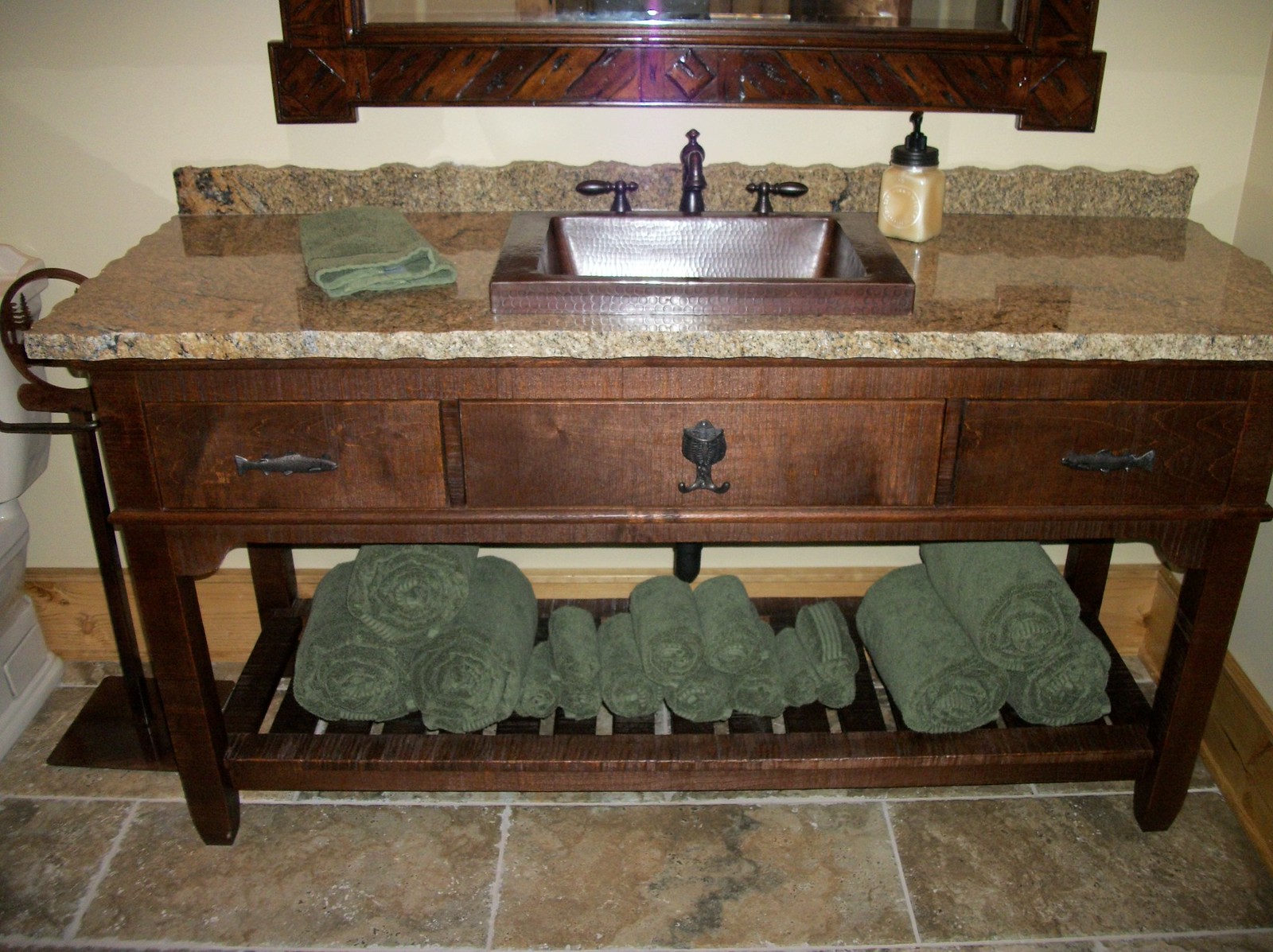The image depicts an opulent upper-class bathroom vanity with a prominent, high-quality herringbone-framed mirror crafted from what appears to be walnut or cherry wood. The visible lower portion of the mirror adds a touch of elegance with its rich, wooden texture. Below the mirror, the countertop is a striking slab of brown marble with specks of gray and other nuanced colors, featuring refined scalloped edging.

The sink is notably elevated above the vanity surface, offering a unique aesthetic. It has a seemingly wooden basin, expertly shellacked to prevent water damage and rot. The sink is complemented by dark bronze metal handles on either side and a matching spigot in the center, enhancing the luxurious feel.

Atop the sink, a neatly folded green towel sits beside a large mason jar-sized soap dispenser in cream color with a black lid. The vanity unit includes three drawers; the left and right drawers are adorned with knobs shaped like fish facing each other. The middle drawer, however, features a double-sided hook for hanging towels, suggesting it might not be a functional drawer but rather a decorative or alternative storage space.

Beneath the vanity, an open section reveals a single dark bronze pipe, with a neatly arranged stack of towels rolled up in a manner resembling cinnamon rolls, adding a cozy touch to the sophisticated setup. Off to the left, a white toilet, which is notably less elaborate than the sink, is accompanied by a fancy toilet paper holder, though devoid of toilet paper. The bathroom is floored with large ceramic tiles, accentuated by fairly white grout lines.

Overall, the image suggests a high-end bathroom setup, with significant investment in the sink vanity's luxurious design and materials, reflecting upper-class tastes and attention to aesthetic detail.